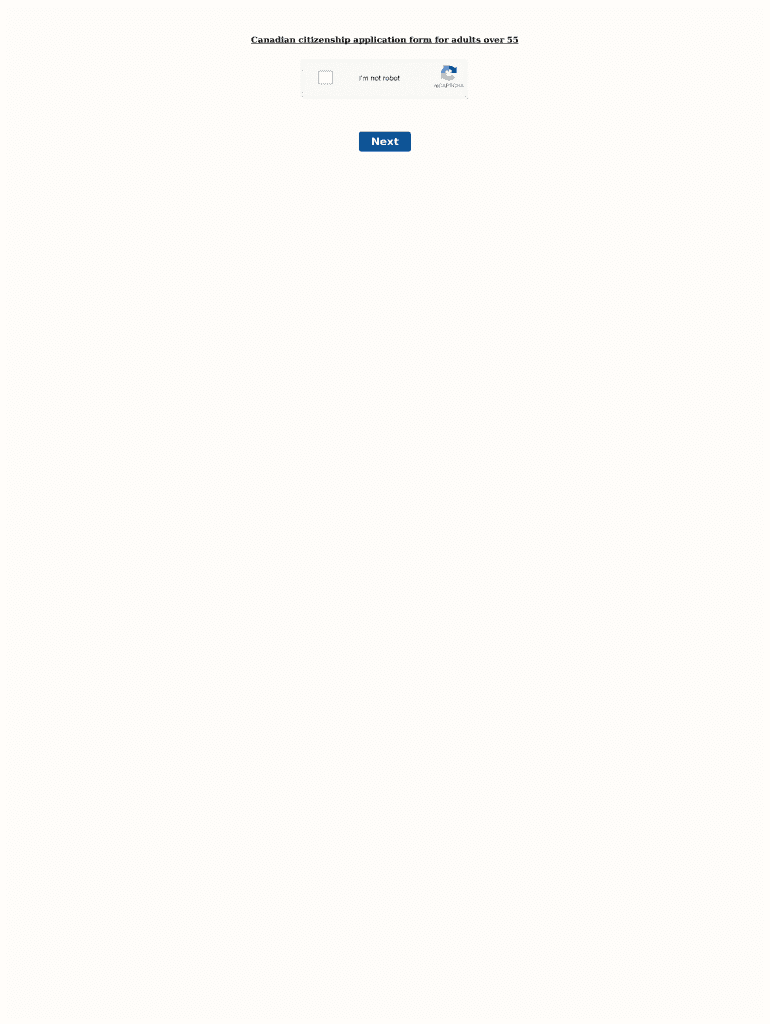Screenshot featuring a minimalistic white background with scattered, mostly illegible text. The legible portion includes the words "Canadian," "price now," "free," "adult," and "max" in black font. Additionally, there is an unchecked CAPTCHA box accompanied by the statement "I am not a robot" alongside the CAPTCHA logo. Below this is a dark blue button which potentially reads "Next."